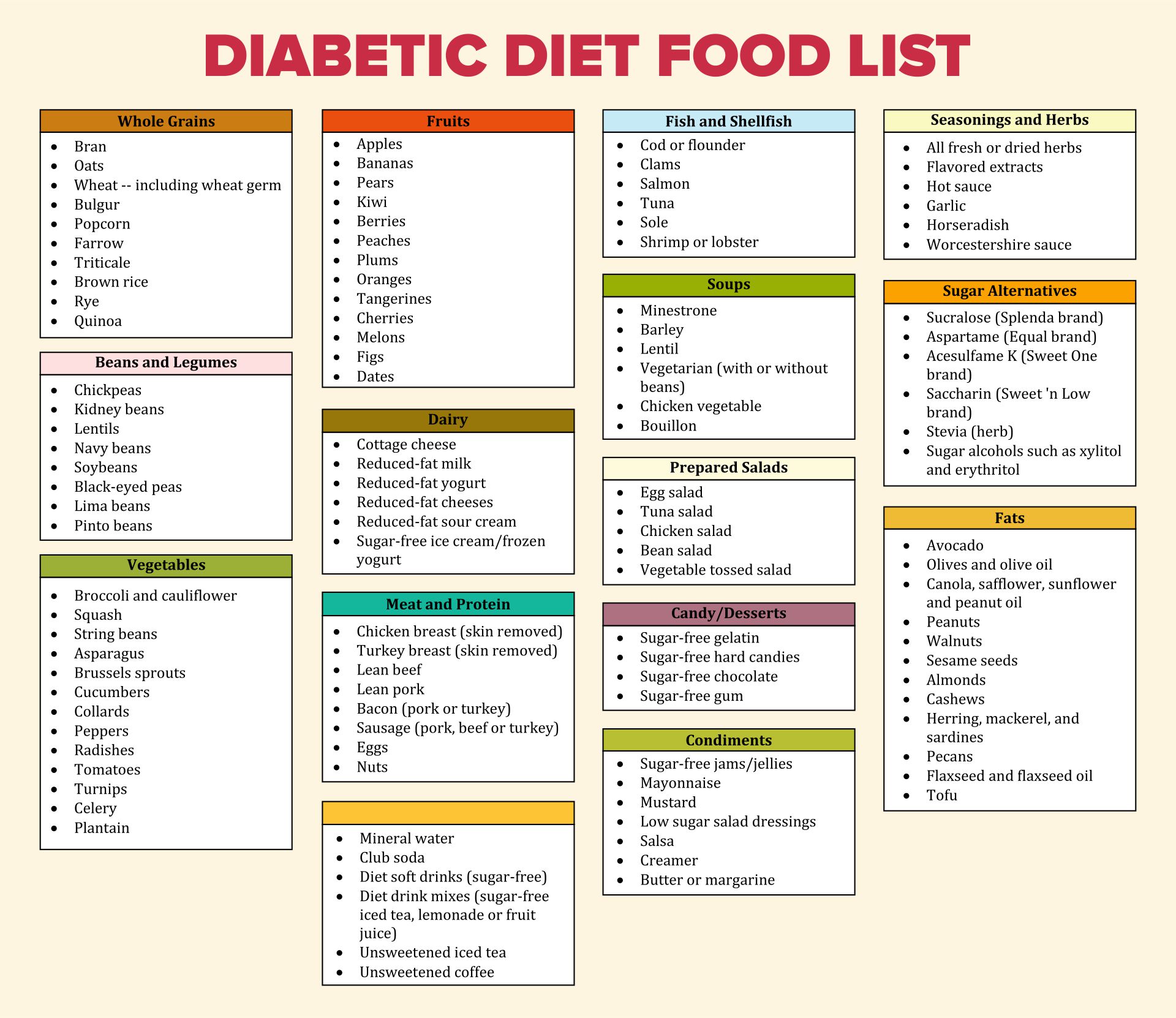The image is a detailed square chart labeled "Diabetic Diet Food List" in large red letters at the top center. The chart is organized into multiple white rectangles, each with a colored heading and black text outlining specific food categories. The headings, written in black, include various categories such as whole grains, fruits, vegetables, dairy, meat and protein, fish and shellfish, beans and legumes, condiments, seasonings and herbs, prepared salads, soups, candy and desserts, sugar alternatives, fats, and beverages. For example, the green box labeled "Condiments" lists diabetic-friendly options, while the "Whole Grains" box includes foods like bran, oats, wheat, popcorn, and farro. Each category contains a detailed list of foods suitable for a diabetic diet, such as broccoli, cauliflower, and asparagus under vegetables; apples, bananas, and berries under fruits; and salmon, tuna, and shrimp under fish and shellfish. The chart provides a comprehensive selection of foods, ranging from 4 to 15 items per category, to guide individuals in making healthy dietary choices.